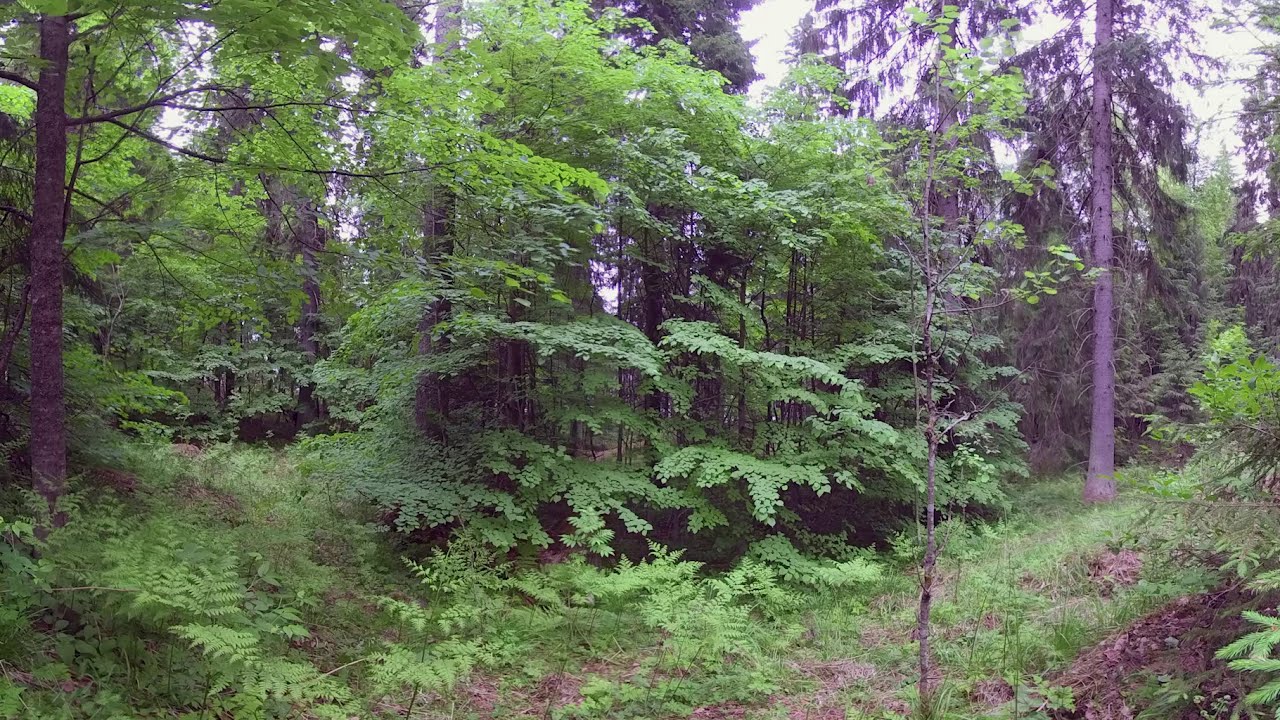This image captures a dense, temperate forest scene, characterized by a muted green palette likely enhanced by a lens filter, which subdues the vibrancy of the foliage. The day appears overcast, limiting direct sunlight, although there is a minor opening in the sky at the top right corner, suggesting some light filtration. The foreground and mid-ground are peppered with ferns, wild grasses, and patches of dirt and mulch, indicative of a natural forest floor. Deciduous trees dominate the scene, with some hints of evergreens in the background. Many trees exhibit signs of decay or death, with one notable tree on the right side of the frame bearing predominantly brown, withered branches. Despite this, the greenery, especially the ferns and grasses, is visibly thriving. The lack of discernible paths suggests an untamed stretch of woodland, providing a serene, albeit slightly somber, snapshot of nature.